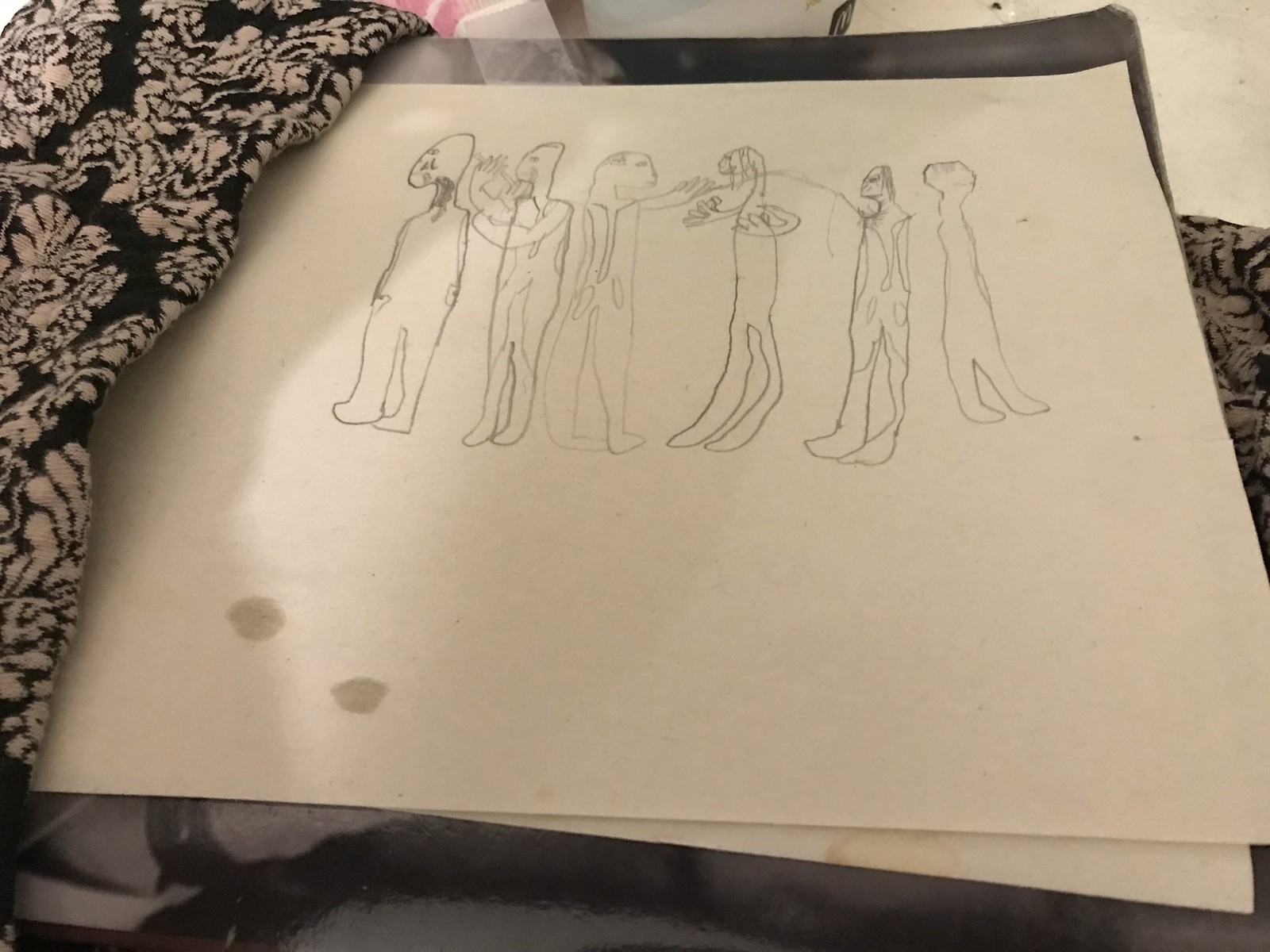This image showcases a pencil sketch on a piece of white construction paper, oriented landscape. The sketch, likely done by a young artist, attempts to depict six human figures. Despite the rough nature of the drawing, it's clear that the artist used only a single pencil, creating a monochromatic gray illustration. The sketch is positioned mostly overhead and slightly forward, indicating that the paper lies flat on a surface. To the left of the paper, a towel or blanket is visible, though its precise nature remains unclear. Additionally, there are other indistinguishable items placed beneath the piece of paper, adding context to the setting in which the drawing was created.